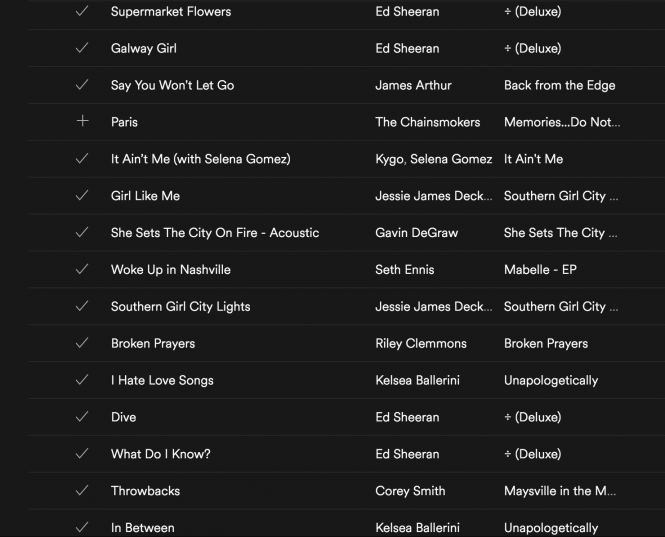A detailed view of a playlist or song list is presented in a landscape orientation with a black background. A thick black margin with no content is situated on the left side of the image. The list comprises 15 songs, formatted into three columns displaying the song title, artist, and album. Each entry is marked with a check, except for one which is indicated by a plus symbol, possibly denoting a newly added track or a song currently being listened to.

1. "Supermarket Flowers" - Ed Sheeran
2. "Galway Girl" - Ed Sheeran
3. "Say You Won't Let Go" - James Arthur from the album "Back From the Edge"
4. "Paris" - The Chainsmokers from the album "Memories... Do Not"
5. "It Ain't Me (with Selena Gomez)" - KYGO & Selena Gomez from the album "It Ain't Me"
6. "Girl Like Me" - Jessie James Decker from the album "Southern Girl City"
7. "She Sets the City on Fire (Acoustic Version)" - Gavin DeGraw from the album "She Sets the City"

This selection exemplifies a diverse blend of pop and contemporary hits, featuring both top-charting artists and notable albums. The clear organization provides seamless navigation through the playlist, enhancing the listening experience.